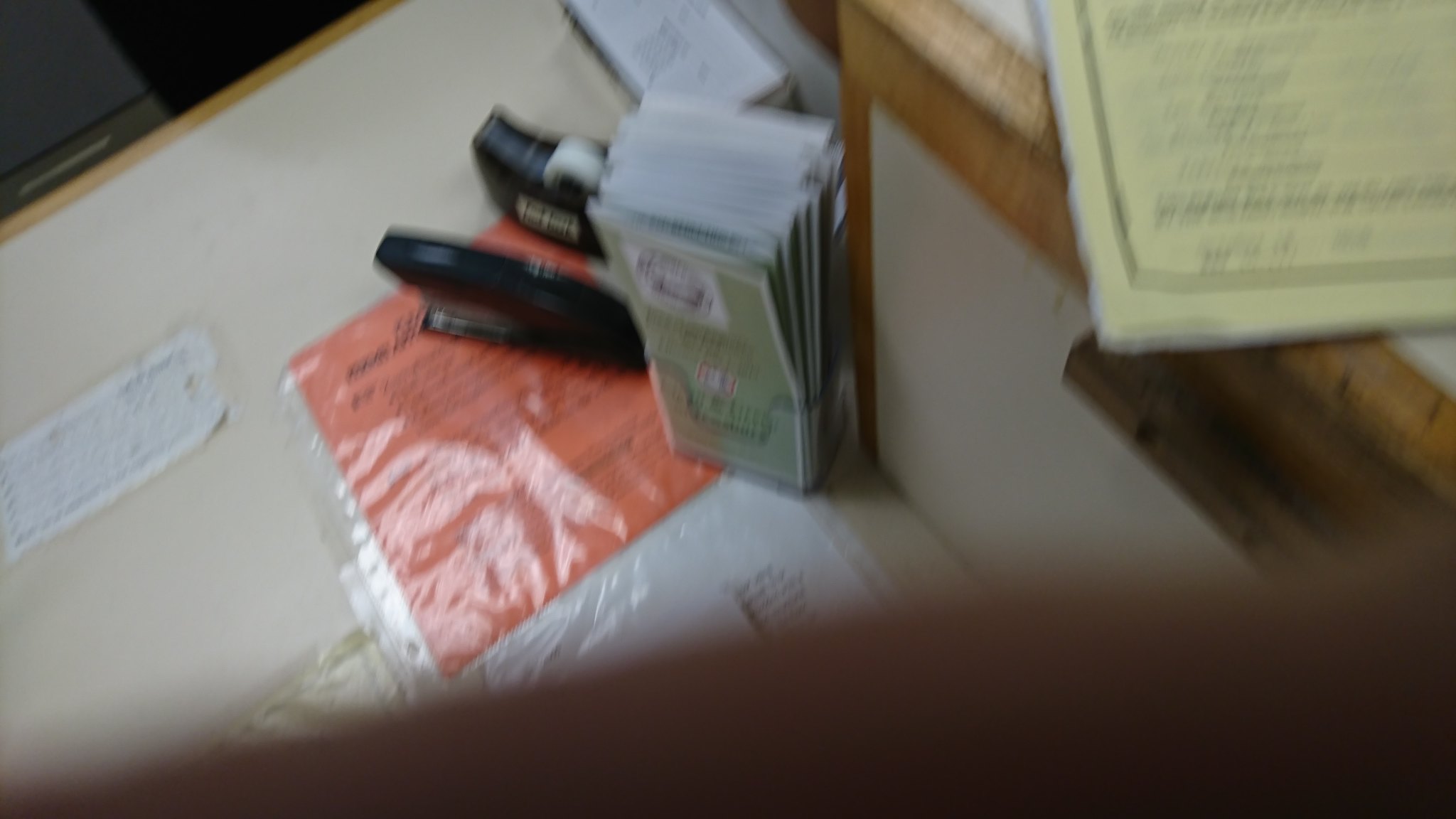On the right side of the image, there is a white menu displaying some text. Adjacent to the menu is a neat stack of brochures, partially revealing the edge of a box, and additional brochures containing various pieces of information. The scene is set on a white table, where a white rectangular card with some text is also placed. Nearby is an orange rectangular card with black text, alongside some type of reflective material. A stapler is present on the table, and above this setup is a roll of tape on a dispenser, complete with its inner roll visible.